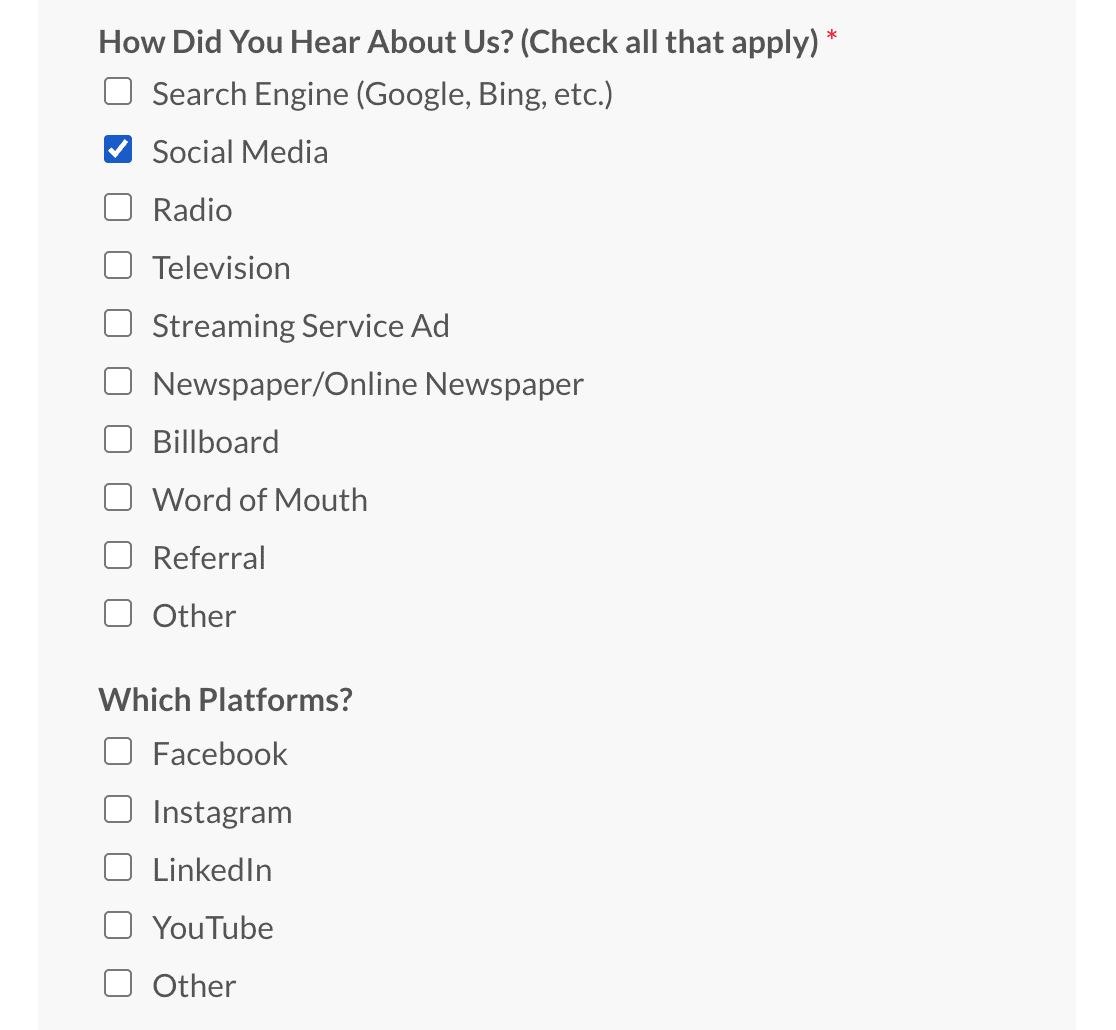This image depicts a survey form with a light gray background. At the top, there is a bold, black heading that reads, "How did you hear about us?" followed by a question mark. Beneath this, in parentheses, it says, "Check all that apply," accompanied by a red asterisk indicating a mandatory field.

The form includes a series of checkboxes arranged in a list. The options are as follows:
- Search Engine (Google, Bing, etc.)
- Social Media (with this particular checkbox filled in blue and marked with a white checkmark)
- Radio
- Television
- Streaming Service Ad
- Newspaper/Online Newspaper
- Billboard
- Word-of-Mouth
- Referral
- Other

Following this list, there is another bold heading, "Which platforms?" with a question mark. Below this are additional checkboxes next to the following options:
- Facebook
- Instagram
- LinkedIn
- YouTube
- Other